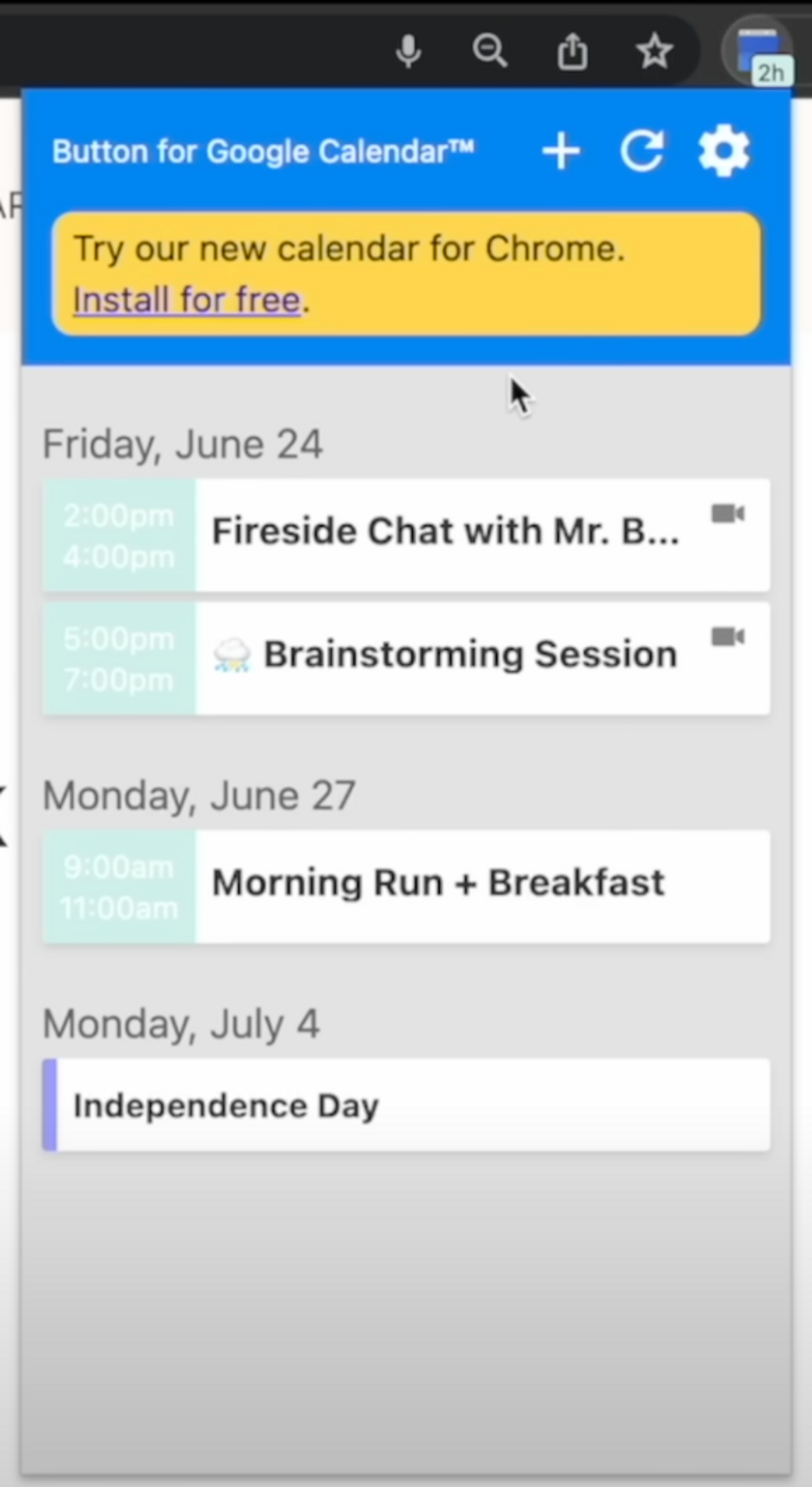Here is a more detailed and cleaned-up caption for the described image:

---

A screenshot of a cell phone displays an interface filled with various icons and textual elements. Across the top of the screen, there are icons for a microphone, a magnifying glass (search), an upload button, and a favorites button. Below these icons, the text "button for Google Calendar" appears, accompanied by additional icons: a plus sign for adding events, a reload button for refreshing the calendar, and a sprocket icon for accessing settings.

The next section of the screenshot features a highlighted yellow field containing a promotional message that reads, "Try our new calendar for Chrome, install for free," with the phrase "install for free" rendered as a clickable hyperlink. A black mouse pointer is located just below this text, indicating user interaction.

Further down the screen, the calendar displays several scheduled events:

- **Friday, June 24th:**
  - **2 p.m. to 4 p.m.** - Fireside chat with Mr. B...
  - **5 p.m. to 7 p.m.** - Brainstorming session

- **Monday, June 27th:**
  - **9 a.m. to 11 a.m.** - Morning run with breakfast

- **Monday, July 4th:**
  - Independence Day

The entire calendar view is set against a gray background, framing the details in a straightforward, user-friendly layout.